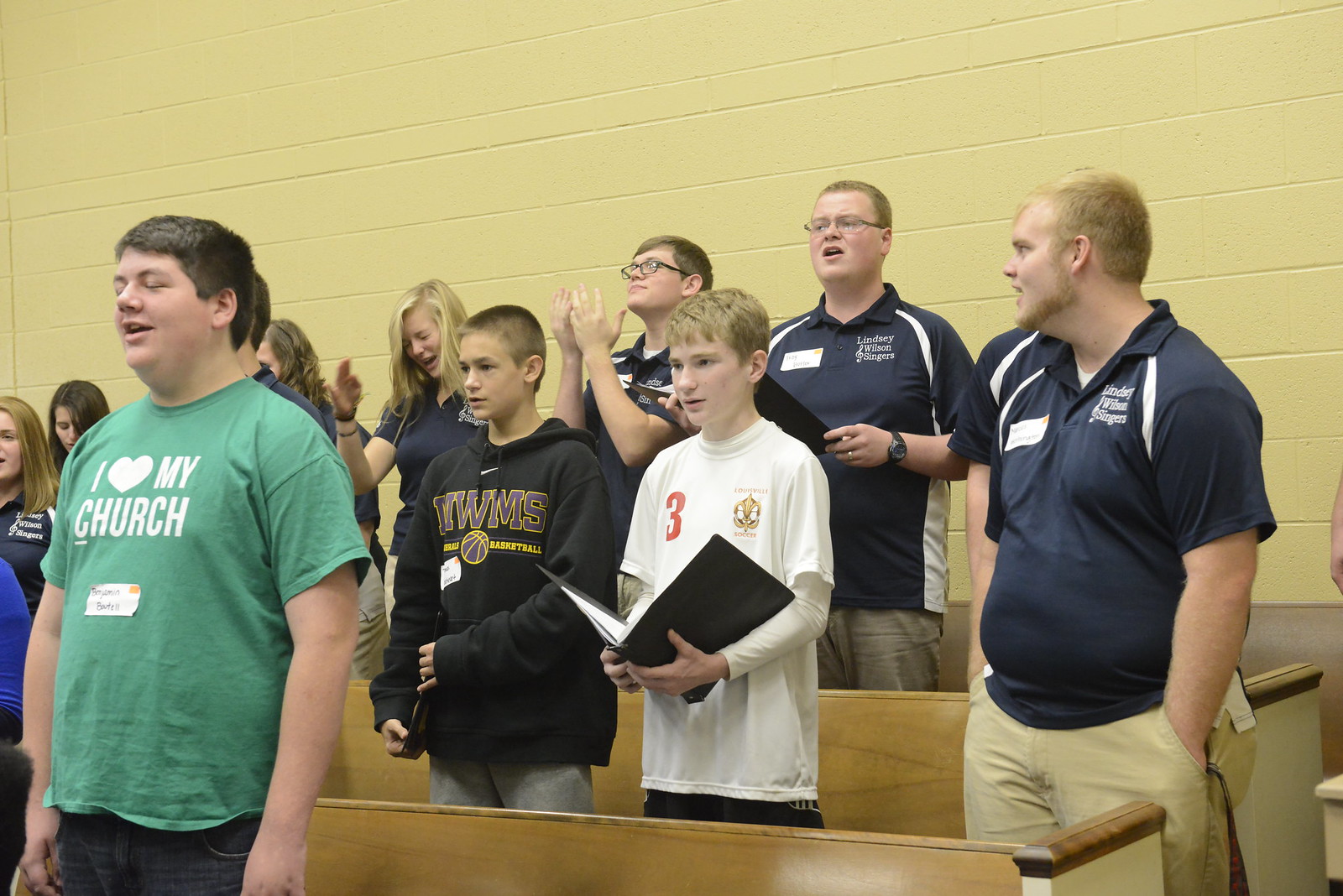The image captures a group of approximately 10 to 15 teenagers standing in rows of wooden pews that suggest the setting is a church. Behind them is a cinder block wall painted yellow. The teens, male and female of various ages, are all holding black choir books filled with sheets of music or lyrics, and their open mouths suggest they are singing or reciting something. Their attire is casual and varied, with at least one boy prominently wearing a green shirt that reads "I love my church" or "I heart my church." Other notable items of clothing include a black hoodie with the letters "WMS" and a t-shirt over a long-sleeve shirt with "three" printed on it. Amidst this diverse group, a few teens wear dark blue polos, adding to the variety in their casual wardrobe.